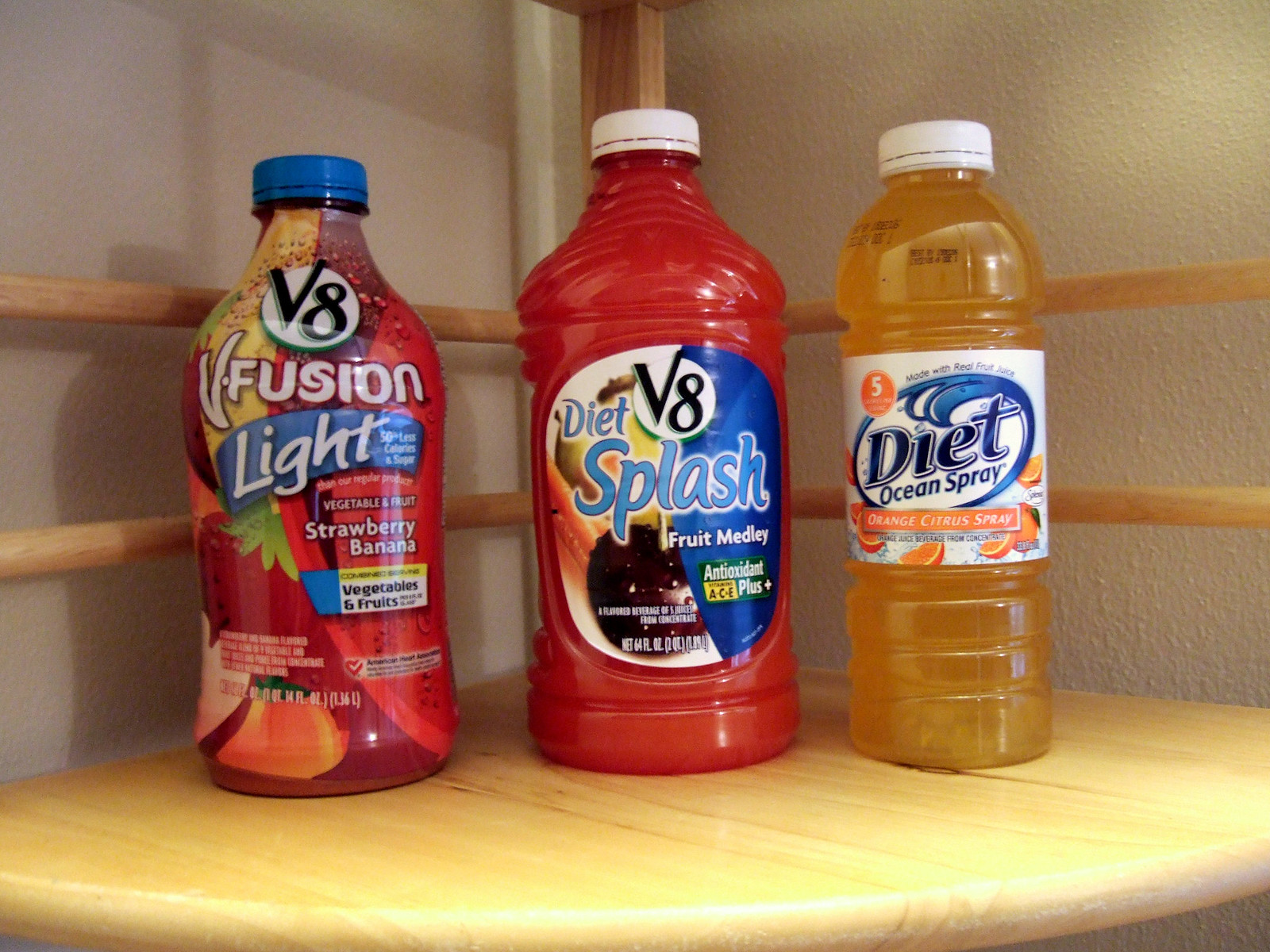This image depicts a wooden corner shelf designed to fit neatly into the intersection of two walls. The shelf has a back support structure made of wooden crossbars, providing both stability and a decorative touch. Resting on the shelf are three beverage bottles, each distinctly different in appearance and size.

On the left, there stands a vibrant, approximately 64-ounce bottle of V8 Fusion Might, notable for its bright and eye-catching colors. In the center, there's a 64-ounce bottle of Diet V8 Splash Fruit Medley, which is a reddish-orange color with a label featuring a multitude of hues. To the right, a smaller, clear 20-ounce bottle of Diet Ocean Spray reveals its orange contents, and its label is adorned with white, orange, and blue elements.